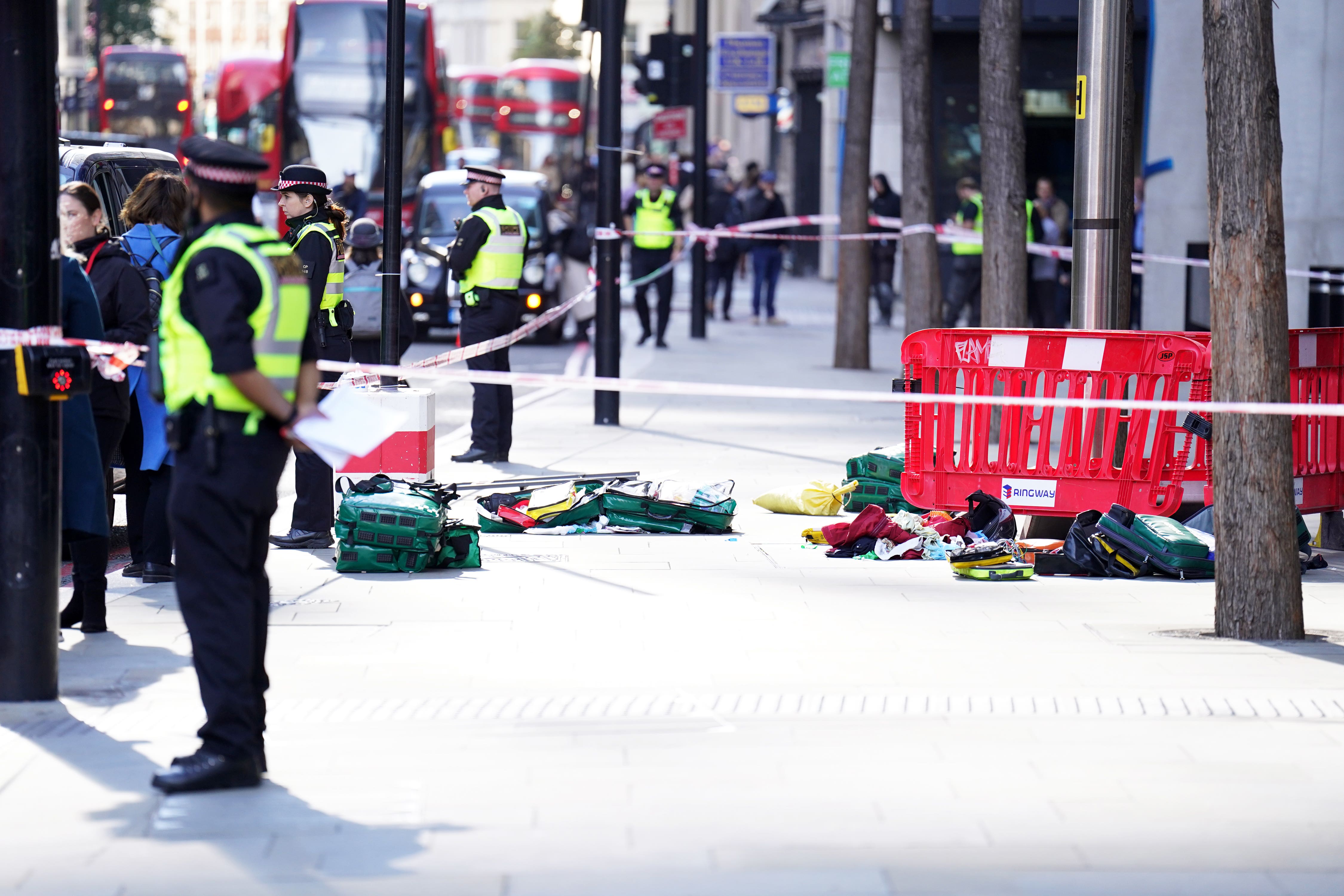A detailed photograph captures a scene involving a group of police officers standing around a cordoned-off area on a city sidewalk. The outdoor setting features a sidewalk lined with black poles and lush trees on the opposite side. The officers have used white tape to cordon off the space, meticulously wrapping it around the trees and poles to secure the perimeter. The police are stationed at various points around the boundary, facing outward with their backs to the enclosed area, maintaining a vigilant presence. Within the tape-enclosed zone, a notable red container or a set of red dividers stands out, bearing a conspicuous white label that reads "Ringway." Strewn across the ground inside the restricted area are numerous open cases and bags that resemble luggage, contributing to the scene's sense of urgency and investigation.